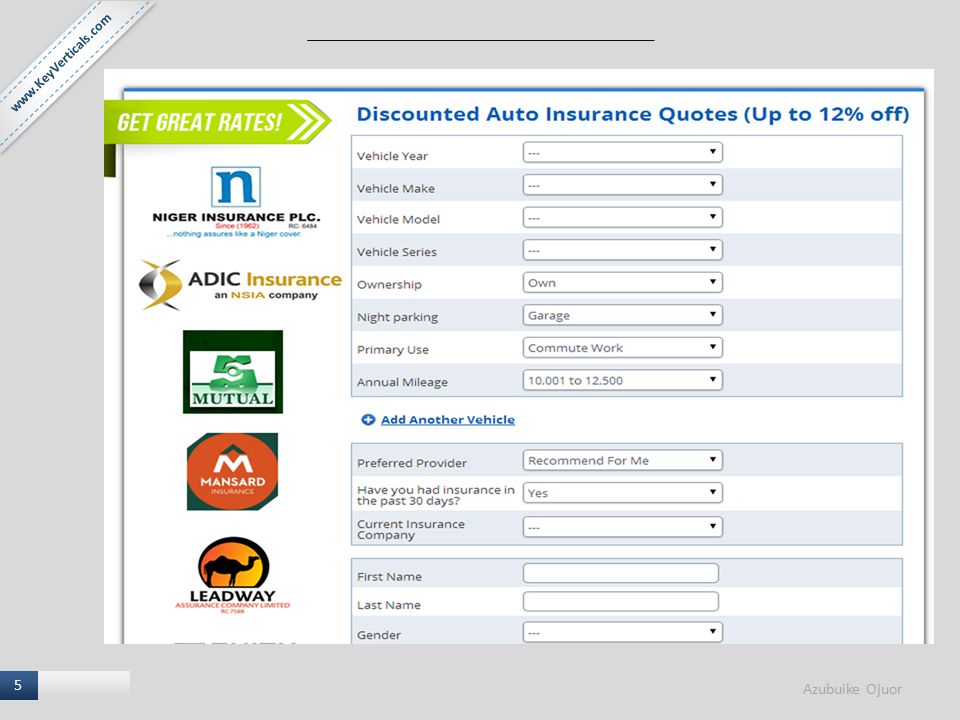A detailed screenshot of an old-fashioned web page is overlaid onto a graphic design with a medium gray background. In the top left corner, a 45-degree stripe features blue dashes on the top and bottom edges, with blue text that reads "www.keyverticals.com" overlaying the stripe. Across the center top, a thin black line spans about the middle third of this section. In the bottom left, there's a gradient gray box, next to which is a gradient dark blue box displaying a large white number five.

In the bottom right corner, gray text states "Azabuike, au jour." The overlaid web page has a white background, with a prominent header in blue text reading "Discounted auto insurance quotes up to 12% off." Below this header, there are multiple sections with alternating white and gray lines. Each section contains a label and an empty drop-down box, unless stated otherwise. 

From top to bottom, the sections are labeled:
- Vehicle Year
- Vehicle Make
- Vehicle Model
- Vehicle Series
- Ownership: Own
- Night Parking: Garage
- Primary Use: Commute to Work
- Annual Mileage: 10,001 to 12,500 miles

Separating the sections, blue text reads "Add another vehicle."

Below this, another box with alternating lines contains further sections:
- Preferred Provider: Recommended for me
- Have you had insurance in the past 30 days? Yes
- Current Insurance Company (empty drop-down box)